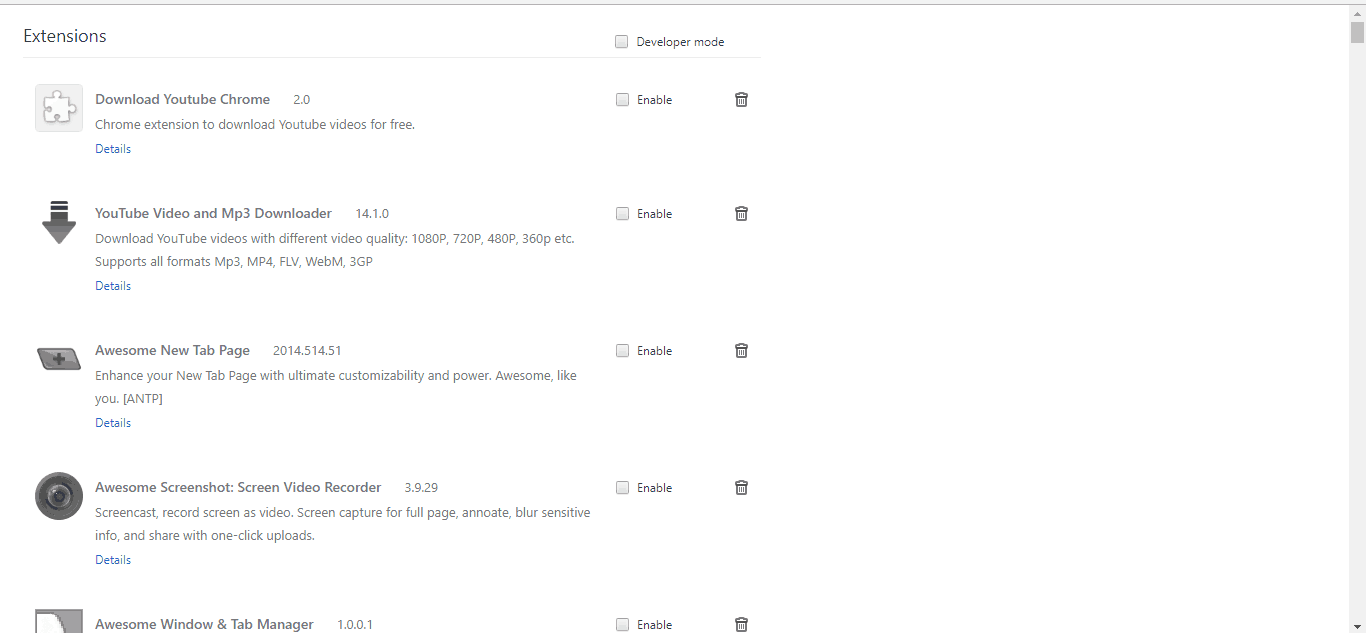A detailed screenshot of the Chrome web browser is presented, specifically showcasing the "Manage Extensions" page. The interface prominently displays the title "Extensions" at the top. Below this, there is a checkbox option to enable "Developer Mode."

The main content area features a list of installed extensions, none of which are currently activated. The extensions listed include:
1. Download YouTube Chrome
2. YouTube Video and MP3 Decoder
3. Awesome New Tab Page
4. Awesome Screenshot Screen Video Recorder
5. Awesome Window and Tab Manager

Each extension entry includes an enable checkbox positioned to the right side, which are all unchecked, and a trash can icon that allows for the deletion of the respective extension.

The layout is utilitarian, with a vertical scroll bar on the far right side, indicating the presence of more content below the fold. The top and bottom of the page are otherwise sparse, providing no additional control elements or widgets.